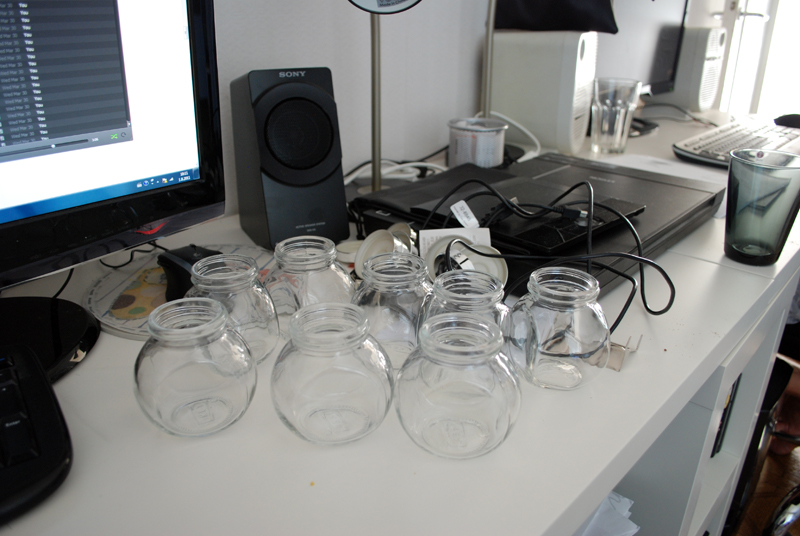This photograph captures a busy and detailed workstation setup against a white wall. Central to the image is a long white desk laden with various items. Prominently featured is a PC monitor, which is turned on, and a corner of a black keyboard can be seen near it. The desk is cluttered with eight round, lidless glass jars, reminiscent of Asian cupping jars with thick rims, which are empty and evenly spaced on the surface. Additionally, there is a black laptop partially obscured by a pencil tablet resting on top of it, along with black cables sprawled across. In the background, a black Sony speaker is positioned next to the monitor. Further along the desk, on an adjacent section, there is another keyboard and a pair of tall white computer speakers. A black cell phone and charger are also visible, contributing to the plethora of electronic devices scattered across the scene.